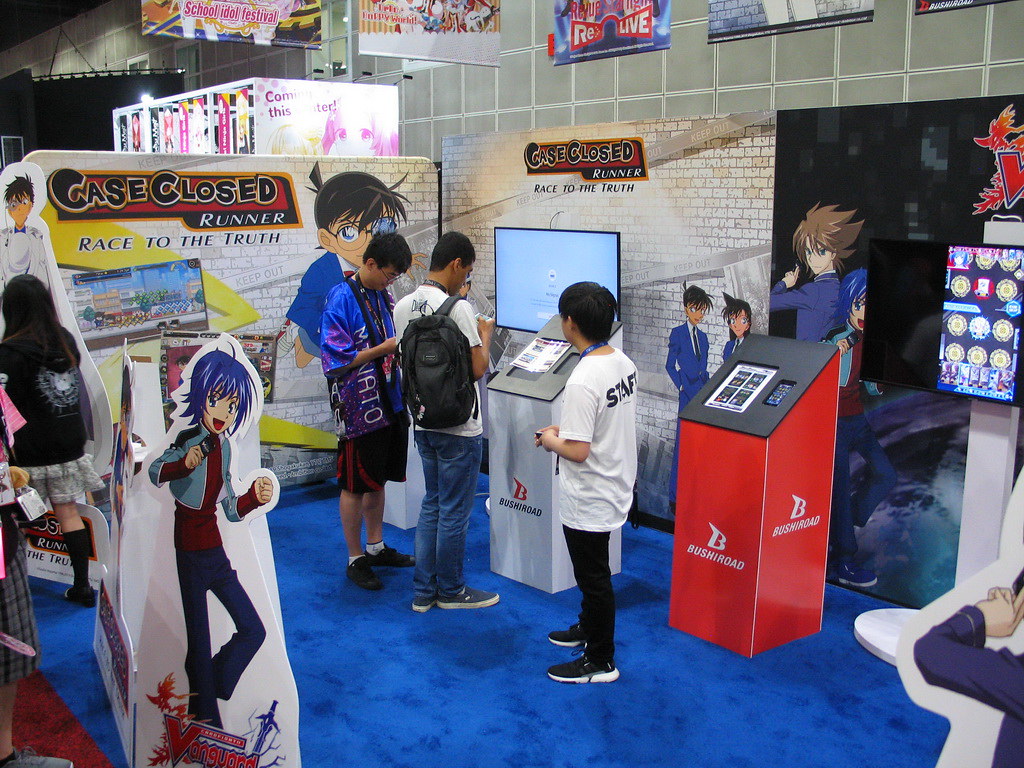The photograph depicts a bustling scene at an anime convention, likely centered around "Detective Conan" (also known as "Case Closed"). The focus is on three teenage boys standing next to a gray podium with a pamphlet on top. Behind them is a television screen mounted on a white brick wall adorned with vibrant graphics and memes touting "Case Closed, Runner, Race to the Truth." The boy on the left wears a blue t-shirt with white text and red graphics, paired with red shorts and black shoes, and dons eyeglasses. The middle boy sports a white t-shirt, a black backpack, blue jeans, and gray shoes. The third boy, possibly an event staff member based on the "staff" label on his white t-shirt, is dressed in black pants and black shoes. The convention floor is covered in blue and features various interactive elements, including cardboard cutouts of anime characters, life-size character statues, and vertical stands with screens, likely demo stations for the event’s featured content. The lively atmosphere is enhanced by the presence of other attendees, including some young girls, and the overall design brims with colorful anime visuals and thematic merchandise.